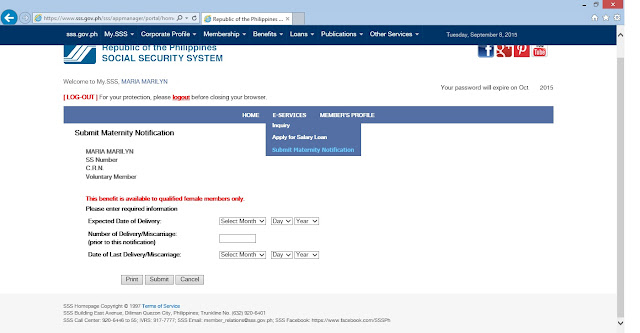This image shows a webpage from the Republic of the Philippines Social Security System (SSS). At the top, a light blue banner spans across the page, displaying the web address to the left, a search bar in the center that reads "Republic of the Philippines...", and a red X icon on the far right to close the page. 

The main content is set against a white background. On the left, in bright blue text, are the words "Republic of the Philippines Social Security System" alongside their logo—a navy blue box containing three white angled lines. To the right of this title are icons for social media platforms including Facebook, Google, Pinterest, and YouTube.

Below this header, in smaller blue text, it welcomes the user with "Welcome to My SSS, Maria Marilyn." Farther to the right, it notes that the user's password will expire in October 2015, and in red text within brackets, the word "Logout" is displayed. Additionally, a cautionary note advises users to log out for protection, with "Logout" highlighted again in red.

A medium blue banner runs horizontally beneath this section. Below the banner, in navy blue text, it says "Submit Maternity Notification." Information about the user is listed underneath: Maria Marilyn, SS Number, CRN, Voluntary Member. In bright red text, a note indicates that the maternity benefit is available only to qualified female members. The remaining section provides space for the user to enter additional data.